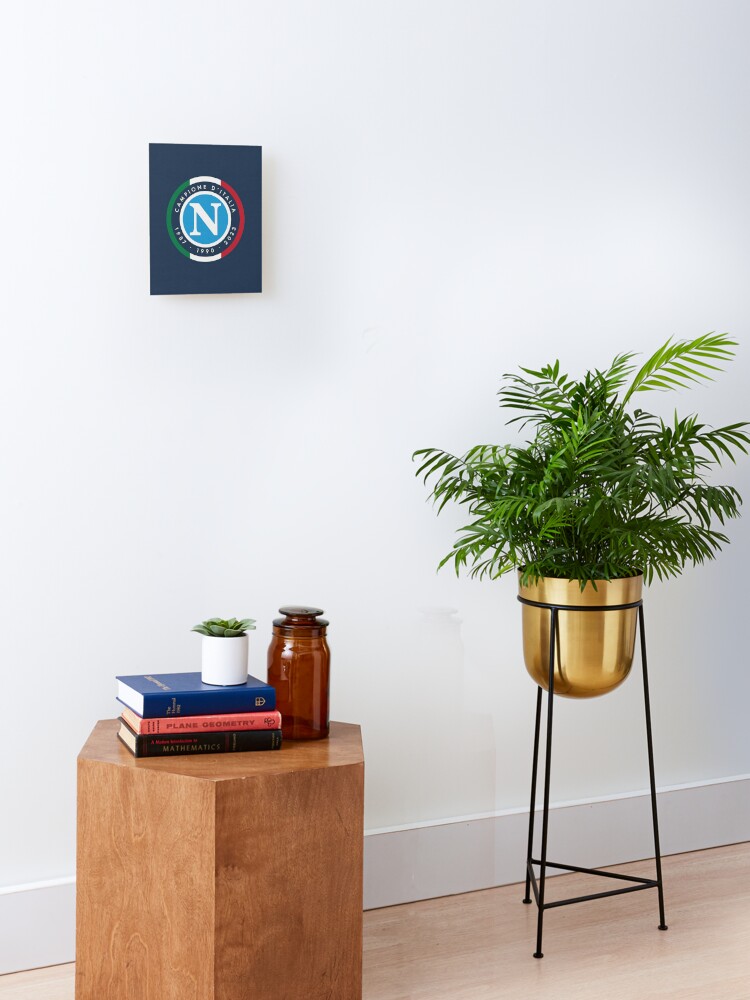This is a photograph of a neatly arranged room with a white wall and a light brown wooden floor. There is a small art piece on the wall; it features a dark blue rectangular background with a central oval bordered by green, white, and red. Inside the oval, a white letter "N" is set against a light blue circle. Towards the left side of the room, a hexagonal wooden table in medium brown stain stands out, displaying three stacked books: the top book is blue, the middle one is a pinkish salmon color, and the bottom one is dark, possibly black. Atop the books, there is a small white planter holding a succulent. To the side of the books, a brown glass container with a lid adds a touch of vintage charm. On the right side of the room, a black triangular plant stand supports a gold planter in which a healthy-looking fern resides, bringing a touch of greenery to the otherwise neutral space.